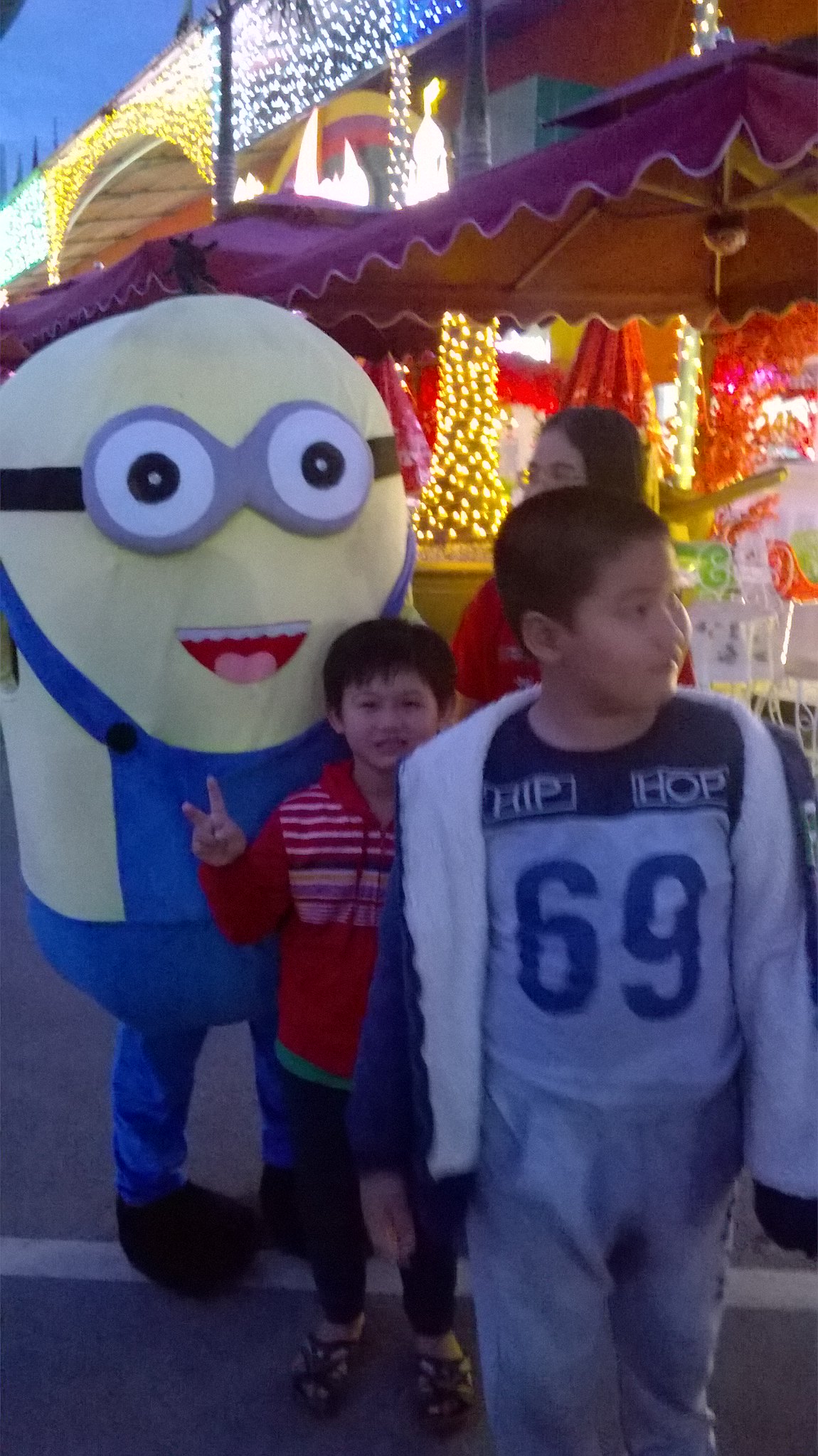In this vibrant and festive photograph, we see two young Asian boys standing outdoors on an asphalt road, possibly at an evening entertainment event or a colorful town celebration. The boy in the front, who appears to be around 9 years old, is wearing a shirt with "hip hop" and the number "69" printed on it, accompanied by gray sweatpants and a blue jacket. Behind him is a younger boy, approximately 5 years old, dressed in a long-sleeved red shirt, black pants, and black sandals, holding up a peace sign with his fingers. The backdrop is lively, featuring bright pink, red, yellow, white, and green lights, festive decorations, and storefronts adorned with sparkly lights and purple umbrellas, suggesting a cold environment. They are flanked by a large character in a costume, likely a Minion from the movie series, dressed in blue overalls and goggles, standing ready to take a picture with the children. A young woman in a red sweater stands behind them, contributing to the joyful atmosphere.